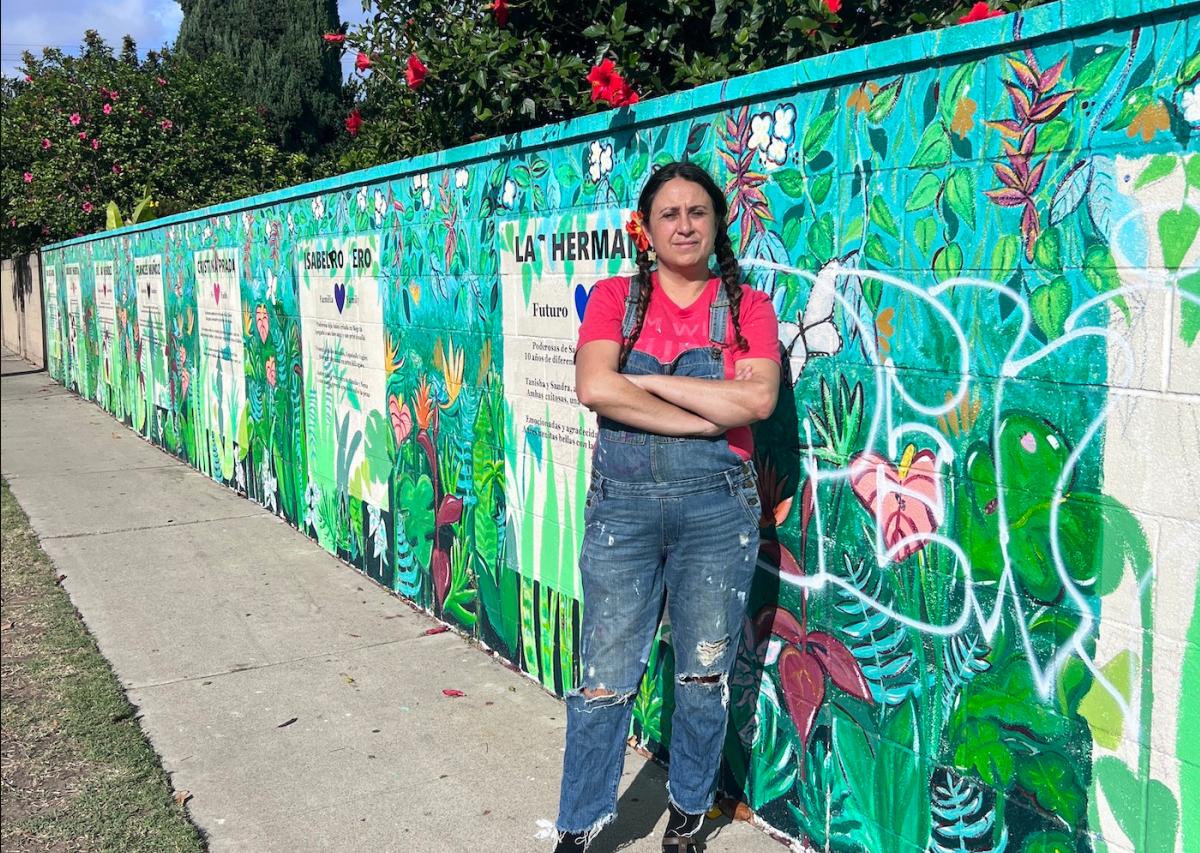In this vibrant image, a middle-aged Mexican woman stands confidently at the center, her arms crossed in front of her chest. She is dressed in distressed denim overalls with holes at the knees and frayed edges, coupled with a red t-shirt. Her long, black hair is neatly parted in the middle, braided into pigtails, with a bright red hibiscus flower tucked behind her ear. She wears black boots that complete her casual yet striking appearance.

The backdrop features a large, artistically painted turquoise blue concrete wall adorned with vivid drawings of tropical plants and flowers. Seven white squares are integrated into the mural, each containing different text, including the phrase "La Herman Futuro," and each accompanied by colorful hearts. Although the exact wording in most squares is indistinct, their presence adds a level of cultural richness to the scene. Above this colorful wall, trees with purple and red hibiscus flowers reach out, adding depth and a lush natural frame to the image. At the woman's feet extends a concrete walking path, while a swath of grass peeks in from the bottom left, reinforcing the setting's blend of urban and natural elements.